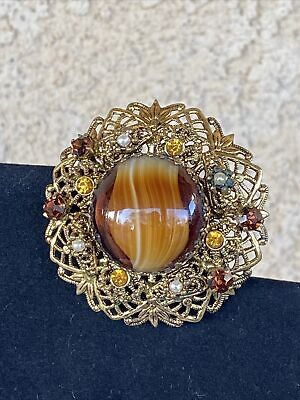This photograph features a close-up of an ornate piece of jewelry, most likely a brooch or a decorative pin, potentially even a ring. Central to the piece is an oval, glass-like gemstone with a shiny, brown and red appearance. Encircling the stone is an intricate, gold, wreath-like design adorned with alternating gems, including small pearls and various colored stones such as gold-toned gems, amethysts, and possibly blue and red emeralds. The composition sits on a blue, soft-textured surface, with a subtle white and gray background that provides contrast and highlights the detailed craftsmanship of the jewelry. No additional context or identifying information is evident in the photograph.